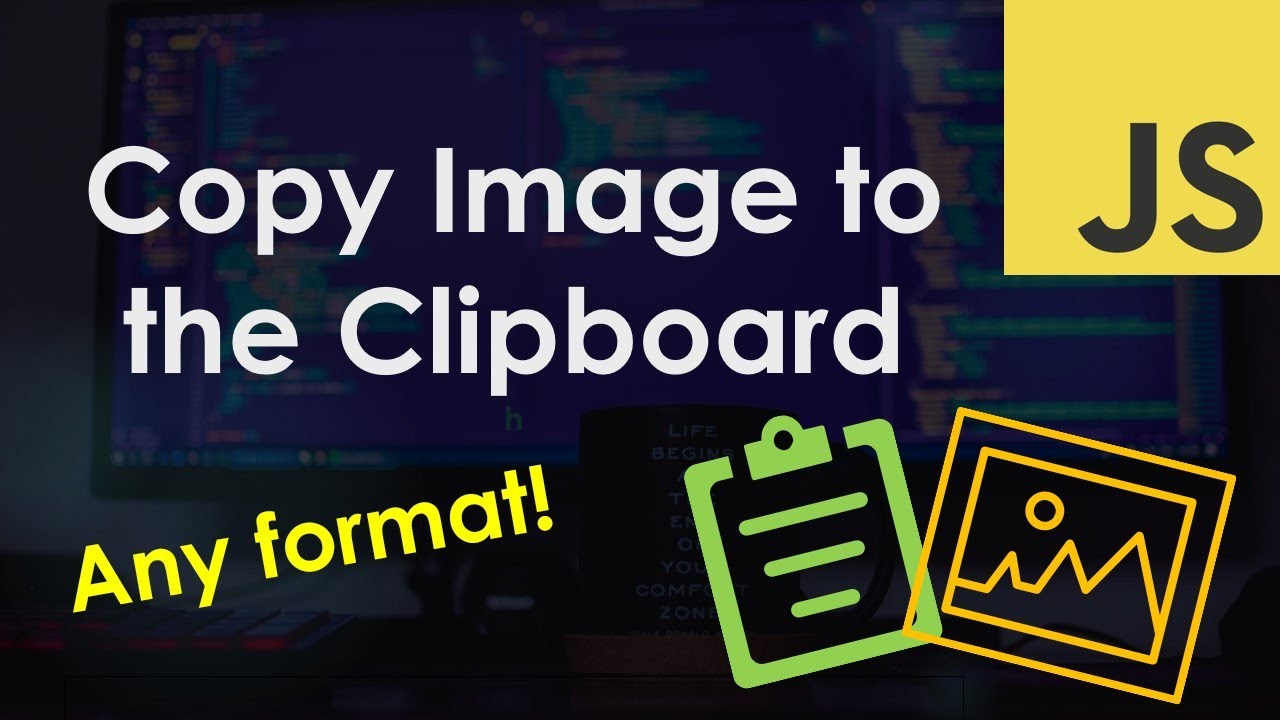The image depicts a computer screen with a dark blue theme and black bezels. In the center of the screen, there is white text that reads "Copy image to the clipboard." Positioned diagonally in the bottom left corner, yellow text states "Any format." In the top right corner, a yellow square contains black letters "JS." At the bottom, two icons are visible: a green notebook-shaped icon on the left, symbolizing the clipboard, and a yellow picture frame-shaped icon on the right, signifying image formatting capabilities. The background behind the computer is blurry but shows a keyboard in the bottom left. Mounted on a board in front of the computer, there is a text that reads "Life begins the time you come out of your comfort zone." The screen displays code, adding to the impression of a workspace setup.